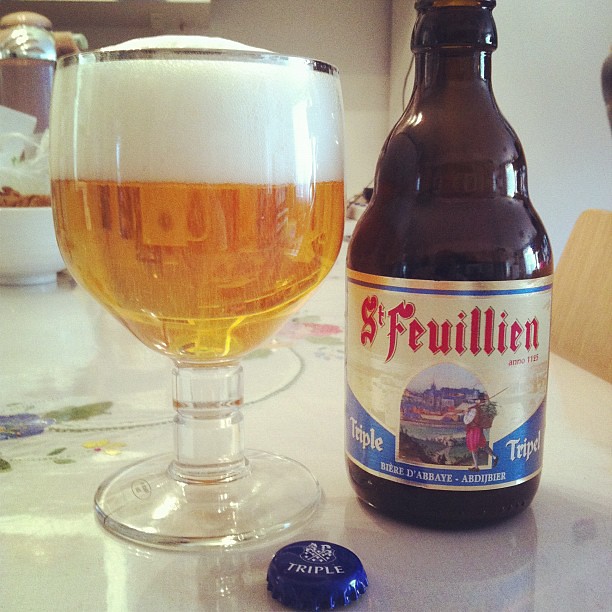This square photograph captures a detailed scene featuring a Belgian beer setup. On the left side, there is a glass goblet filled with beer, which has a thick, white foam head extending slightly above the rim, and a light amber, almost golden liquid filling about two-thirds of the goblet. The goblet itself has a silver rim at the top and a thick stem. 

On the right half, commanding most of the vertical space, is the beer bottle. The bottle is dark brown with a slightly squat shape and a fat neck featuring two layers of shoulders. The label on the bottle prominently displays "Saint-Feuillien" in an old-fashioned Renaissance font in red against a gold background, with the word "Triple" in both English and Belgian spellings on either side. Beneath "Saint-Feuillien," there is an illustrated scene reminiscent of a Renaissance town with a man standing in front.

In the foreground, between the goblet and the bottle, is a blue bottle cap with the word "Triple" in white and a shield logo. The setup is on a tabletop, which appears to have a glass overlay reflecting the objects, hinting at a white tablecloth with flowery patterns beneath. The background contains some indistinct elements, but the primary focus remains on the beer bottle and goblet.